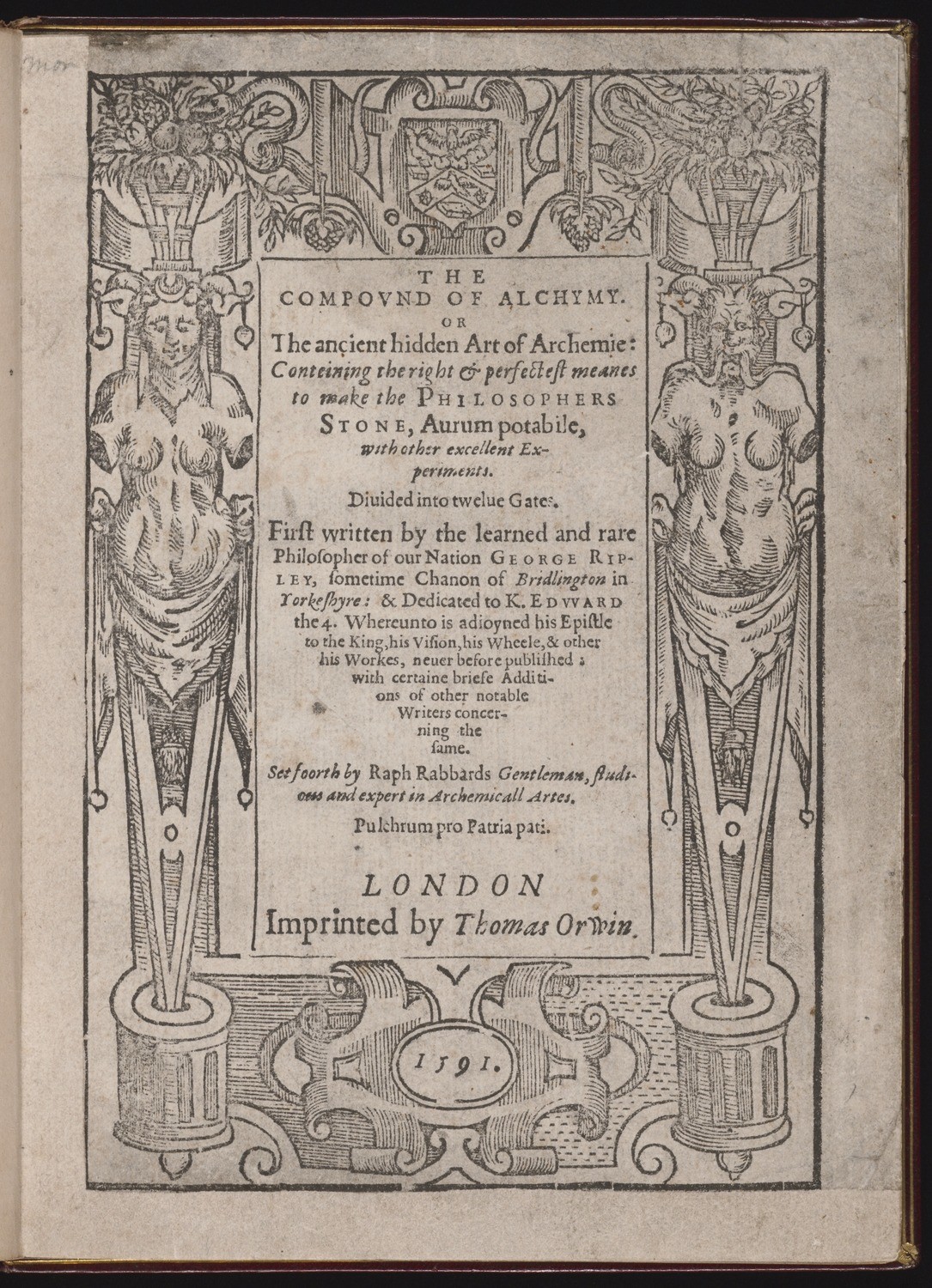This image captures a page from an ancient book, specifically a print from 1591. The vertical rectangular print is bordered on three sides - the top, bottom, and right - by a thin, dark, wooden frame. The background of the print appears to be a light stone or beige color, lending a vintage feel. The central focus of the print is a text block that reads "The Compound of Alchymy, or the Ancient Hidden Art of Archemie," with accompanying intricate details and a paragraph crediting the learned philosopher George Ripley. Below this, it also notes that the text was "Imprinted by Thomas Orwin in London."

Surrounding the text are ornate details, including two armless and legless statues draped with shrouds around their waists. One statue on the left is a bearded man with horns resembling those of a goat or buffalo, while the one on the right is a presumed female counterpart with similar features. Both figures are adorned with ancient decorations, including potted plants and shields, adding to the mystical aesthetic of the page. The craftsmanship suggests it was printed using old printing press methods, and the paper itself reflects an aged, historical appearance, highlighting the age-old practice of alchemy.